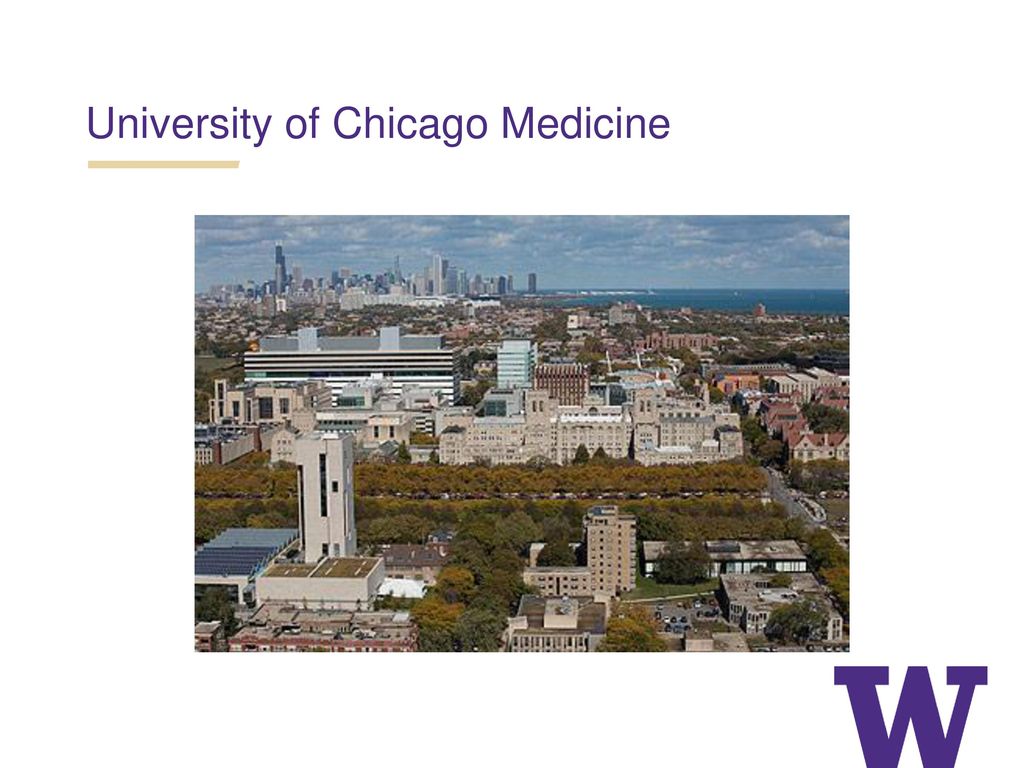The image depicts the University of Chicago Medicine. In the upper left corner, the text "University of Chicago Medicine" is prominently displayed in purple with each significant word capitalized: "University" (capital U), "Of" (capital O), "Chicago" (capital C), and "Medicine" (capital M). Below "University," there is a small space followed by a tan line that extends from under the "U" in "University" to the "I" in "Medicine."

The main body of the image features what appears to be the University of Chicago Medicine campus. The lower right quadrant contains a cluster of buildings, mirrored by another cluster in the lower left. As the image progresses upwards, two rows of trees provide a green canopy that leads to another section of buildings further back. The architectural layout and natural elements create a structured and scenic representation of the campus.